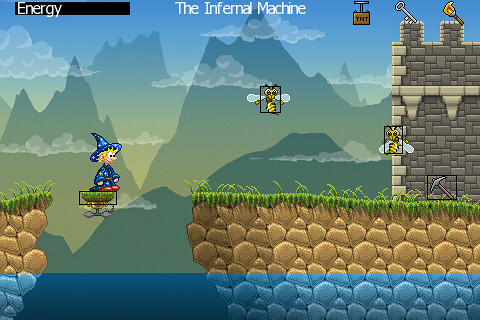This screenshot from the video game titled "The Infernal Machine" features a complex and vibrant scene. The top of the image is dominated by the game's title, "The Infernal Machine," displayed in white letters. A black energy bar is located at the top left, labeled "ENERGY" in white lettering. The gameplay area is split between rocky terrains and sky, with a grassy platform atop a rocky cliff on the left side. Adjacent to this platform is another floating grass platform, equipped with a propeller at its base, carrying a wizard-like character. The wizard, clad in a blue robe adorned with yellow stars, red shoes, a blue pointed hat, and sporting blonde hair and bulging eyes, navigates above a clear blue water feature that sits below the floating platform and cliff faces. 

In the background, wispy clouds drift before rugged mountains, adding depth to the scene. The right two-thirds of the screen show another rocky cliff, a castle wall with parapets, and a pickaxe leaning against the castle base. Additionally, two bees framed in black boxes, suggesting they are enemy units, hover in the sky near the wizard. The top-right corner of the screen displays the user interface elements—a TNT box with a plunger, a grey key, and a torch.

Overall, the image gives a dynamic and lively impression of the game environment, with multiple graphical details and characters that hint at various interactive elements and obstacles for the player to contend with.